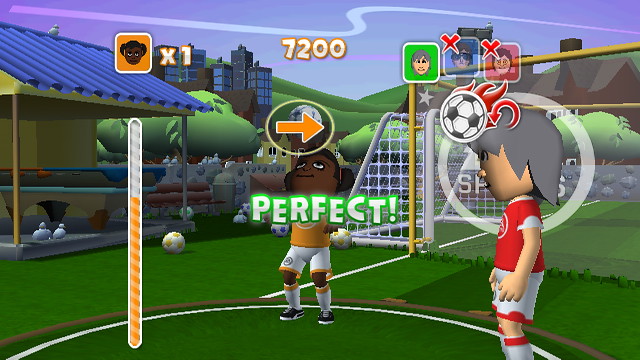The image is a detailed screenshot from a soccer-themed Nintendo Wii video game. Two characters dominate the scene: one on the right, wearing a red sports jersey with white sleeves, white shorts outlined in red, and matching white socks with a red top. This character has light skin and gray hair, reminiscent of Wii Mii avatars. Behind this character is a partial logo comprising of a circle and text, and above them is a fiery soccer ball icon with red flames.

On the left side, there's an African-American girl with her hair bunched up using orange scrunchies. She wears an orange shirt and white shorts with knee-high white socks detailed with orange stripes, and black shoes with white soles. She is looking upwards, likely attempting to hit a soccer ball that is indicated by a yellow circle and an orange arrow. The screen is filled with various game indicators: a horizontal bar that’s over halfway filled with orange, indicating power, and text that reads "PERFECT" in green underneath the arrow.

Above the characters' heads, in the top right corner, are three small, semi-transparent squares featuring avatars, two of which have red X's over them indicating they are out of the game. The third avatar is circled with a white outline and displays the gray-haired character. The game setting shows a field with a soccer goal, a gazebo-like structure with a blue roof to the left, and a cityscape with blue-windowed buildings and green trees in the background.

The screen is rich with color and detail, capturing the dynamic and sporting spirit of the game.